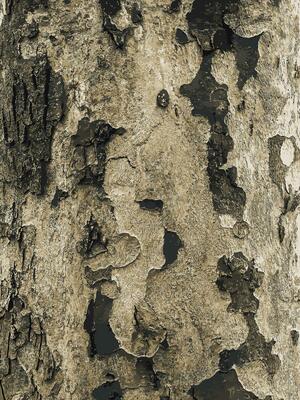The image displays a complex rock formation with a diverse color palette, predominantly featuring shades of brown, a soft tan, beige, and dark gray. The rock seems to be part of an underwater reef with a fossilized appearance, characterized by multiple layers where the underside is darker and the top has a whiter crust. The texture is non-uniform with knobs, straight lines, and formations that perhaps resemble a seahorse. The darker portions appear on the left, transitioning slightly to lighter hues on the right. The rock has intriguing grooves and irregular structures that suggest it has changed over a long period. Imaginatively, the formation might be seen as a one-eyed elephant with a tusk, inside a cavern, interacting with stalactites and stalagmites, adding a whimsical, almost animate quality to the scene.